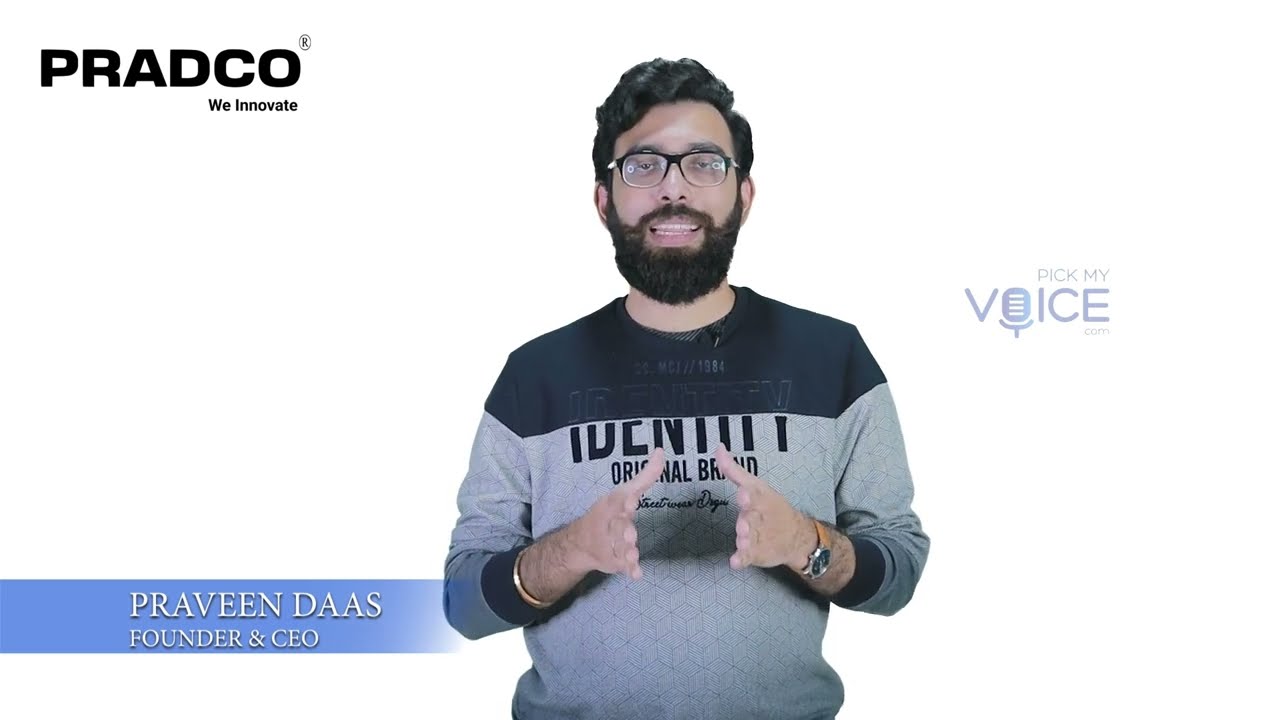This image is a screen grab from a video showcasing a man in his 30s standing in front of a white background, likely a green screen. The man appears to be of Middle Eastern descent, possibly Israeli, with a tan complexion, thick black wavy hair, and a full beard and mustache. He wears black-framed glasses and a gray and dark blue long-sleeve t-shirt that reads "Identity Original Brand," with the sleeves pushed up slightly. He is gesturing with his hands, indicating he is in the midst of speaking. A watch adorns one wrist, while a gold bracelet is on the other. 

Text and logos are positioned throughout the image: in the top left corner, the black text "Pradco, We Innovate"; to the right of the man, a logo that reads "Pick My Voice"; and at the bottom left, within a blue triangular banner, white text that identifies the man as "Praveen Das, Founder and CEO."